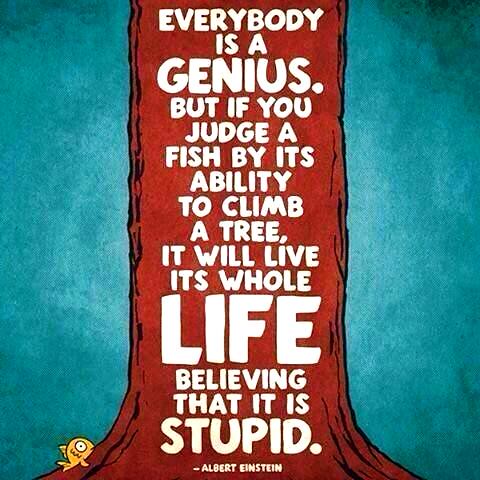The square poster features a captivating illustration with a sea blue and light blue brush stroke background interspersed with hazy white. Dominating the center is a vertically elongated, red-brown tree trunk, drawn in a stylized manner. At the base on the left corner, there's an adorable, round goldfish with a wide white eye, gazing upward towards the text on the tree. The goldfish seems to be attempting to climb the tree, adding a whimsical touch to the scene. The bold white lettering on the trunk reads, "Everybody is a genius. But if you judge a fish by its ability to climb a tree, it will live its whole life believing that it is stupid." The word "life" stands out more prominently. Below the quote, the text is attributed to Albert Einstein, also in white. The overall design merges illustration and graphic typography seamlessly.